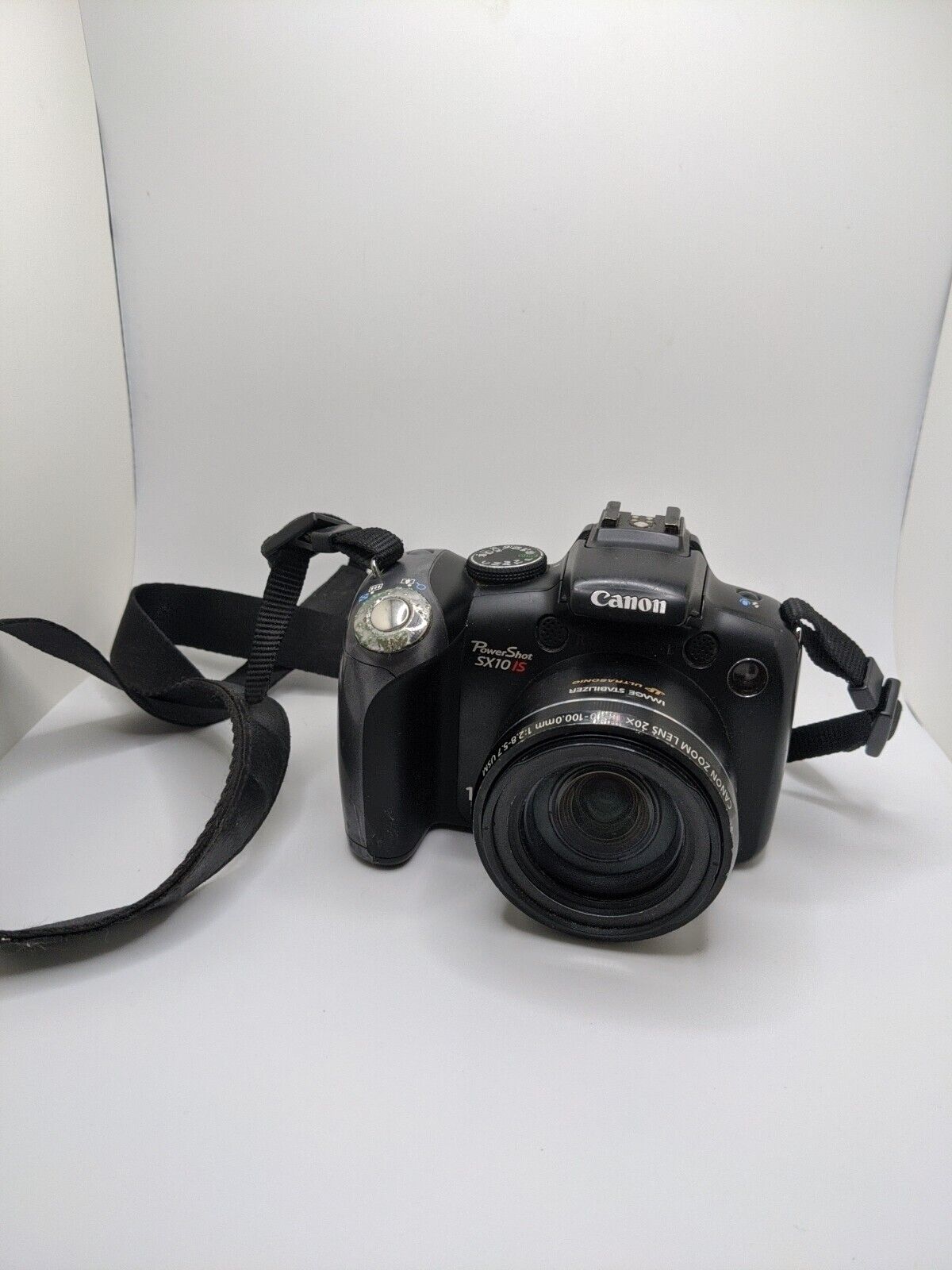This is a detailed photograph of a black Canon PowerShot SX10 camera, capturing it in a minimalist, indoor setting. The camera is placed on a pristine white surface with a matching white backdrop, creating a high-contrast effect that highlights the device's features. The sleek black body of this SLR camera is complemented by a substantial zoom lens, likely marked with "50 millimeters." 

The camera's design includes several noteworthy details: there is a silver knob for the shutter release and a black pentaprism on top, which features the Canon branding. To the left of the Canon logo and just above the lens, "PowerShot SX10" is inscribed. Additionally, it has a hot shoe mount for attaching a flash, a nod to its somewhat vintage style. There are various dials and buttons dispersed around the camera, indicative of its manual settings options. 

A black neck strap is affixed for convenient carrying, looping securely from one side of the camera to the other. This setup, against the white backdrop, suggests a product photography shoot, possibly for listing the camera for sale. The precise and clean composition of the image underscores this focus on showcasing the item’s detailed features visually.